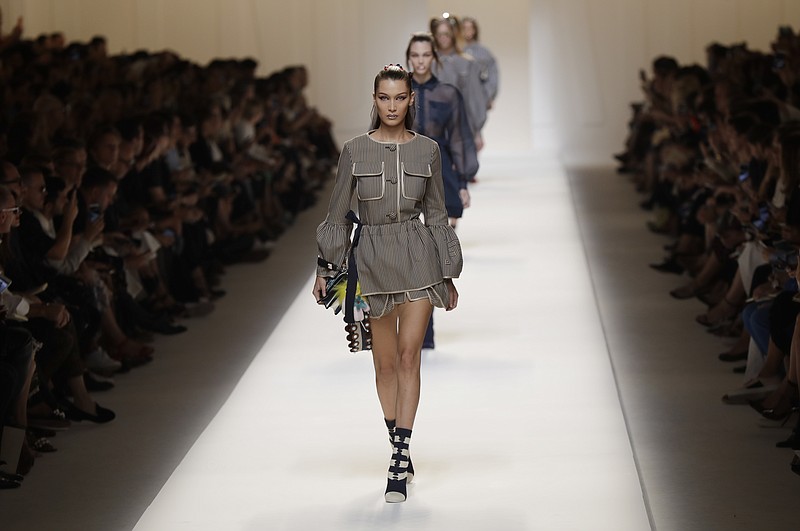This photograph captures a live fashion event, featuring a lineup of female models striding confidently down a brightly illuminated catwalk, showcasing their ensembles. The models, primarily Caucasian with their long hair sleekly pulled back, are dressed in coordinated outfits that consist of long-sleeve blouses featuring breast pockets and very short mini skirts. Their footwear is notably stylish, with each model wearing lace-up boots that rise above the ankles, complementing their overall look. Each model also carries a fashionable purse, adding a touch of practicality to their outfits. The leading model stands out in a gray mini dress accented with white outlines on the breast pockets. In the background, an audience of 30 to 40 people, seated in four or five crowded rows, watches intently, their faces mostly obscured by shadows. The vibrant energy of the festival dedicated to clothing and fashion is palpable in this dynamic scene.